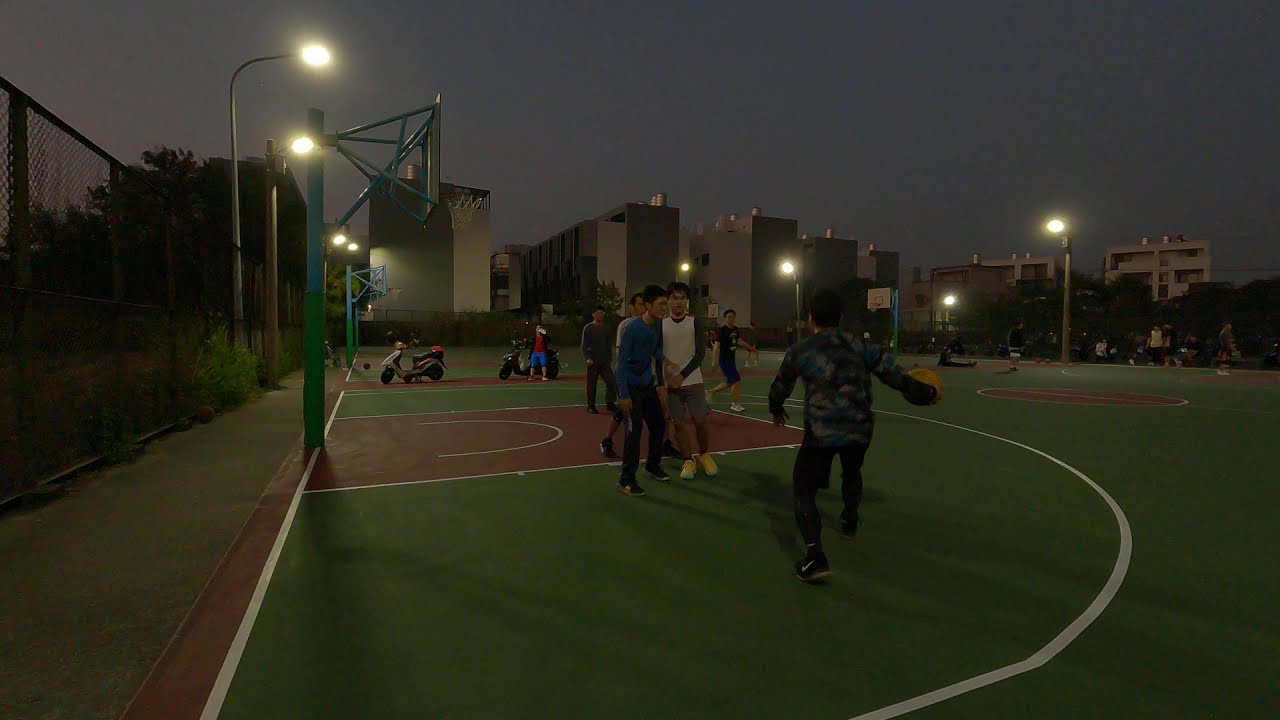In this photograph, set in an outdoor setting during the evening or night, a group of casually dressed individuals is engaging in a lively game of basketball on a green and red court accented with white lines, including clear markings for the three-point and free-throw lines. The scene is illuminated by bright stadium lights, reflecting off the dark gray sky. In the foreground, one player dribbles the ball while several others attempt to guard him, indicative of an active and competitive game. The scene extends to the background where more people can be seen on adjacent courts. On the side of the court, several scooters are parked, with one person standing by a scooter and appearing to drink something. Beyond the court, tall buildings, likely apartment complexes, frame the scene, hinting at the urban environment surrounding this vibrant recreational space.